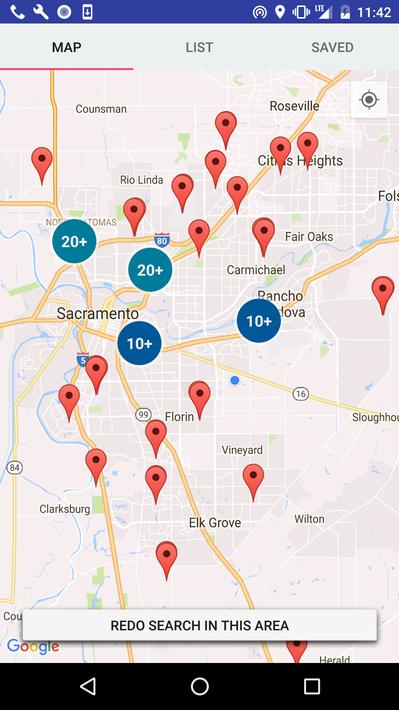This screenshot, taken from a mobile device, displays a detailed view of a map of Sacramento through the Google Maps application. The top section features a blue header with white icons indicative of mobile phone notifications, including a software update availability notification, network connection status, battery life indicator, and the current time. The bottom section contains a black footer with three white navigational buttons: a backward triangle for 'Back,' a circle for 'Home,' and a square for 'Recent Apps.'

The central part of the screenshot prominently shows the map of Sacramento, marked with various red pins indicating specific locations. At the top of the map, there are navigation buttons labeled 'Map,' 'List,' and 'Saved,' with the 'Map' button currently selected, highlighted by a bold pink line underneath. The map is interactive, and at the bottom, there is a white button labeled 'Redo search in this area,' allowing users to refine their search results within the displayed map area.